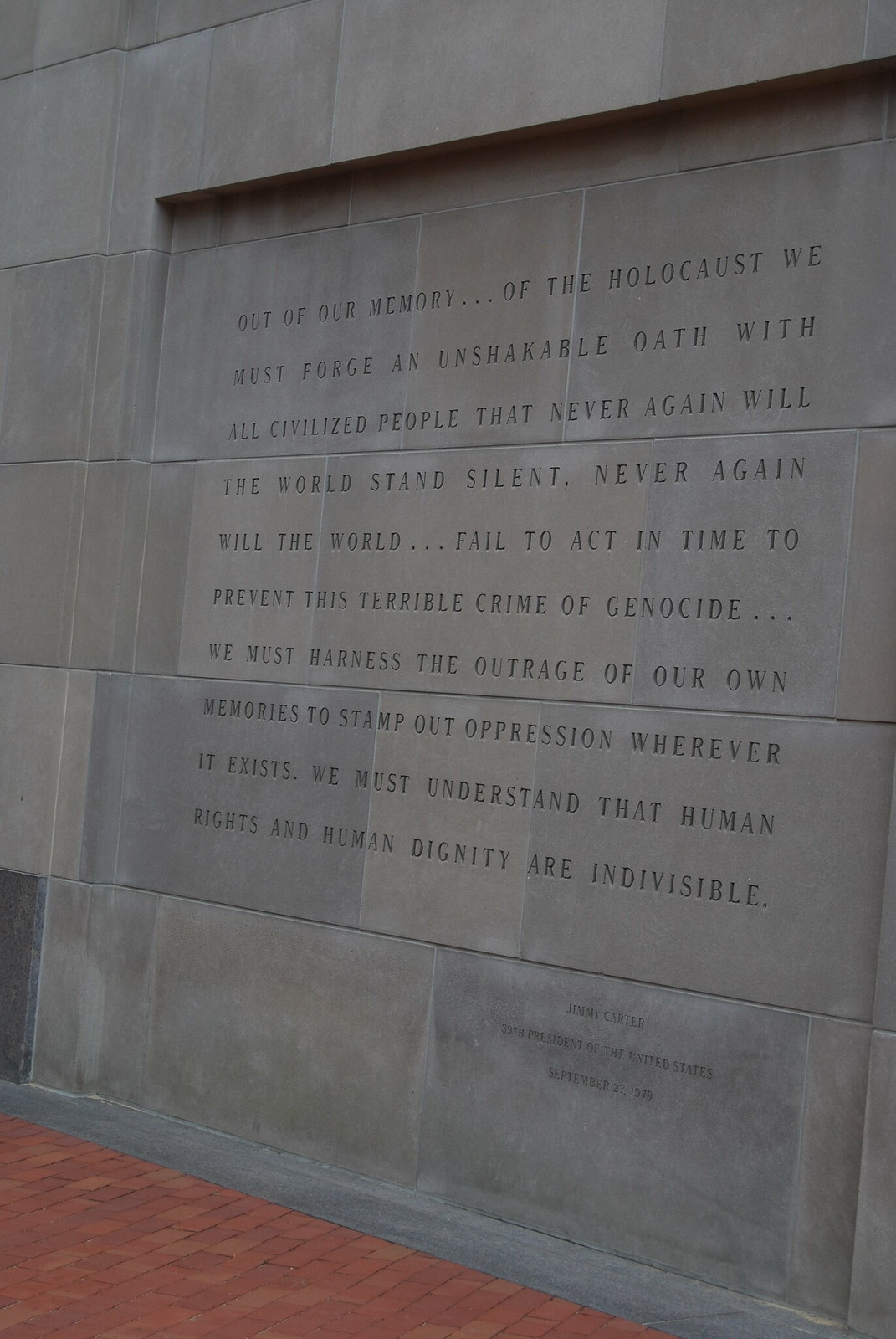The photograph depicts a memorial carved into a large, gray stone wall, made of distinct, rugged stones. The engraved inscription is dedicated to the Holocaust and reads: "Out of our memory of the Holocaust, we must forge an unshakable oath with all civilized people that never again will the world stand silent. Never again will the world fail to act in time to prevent this terrible crime of genocide. We must harness the outrage of our own memories to stamp out oppression wherever it exists. We must understand that human rights and human dignity are indivisible." Below this poignant message, there is a smaller text that is unreadable. In the foreground, the path is made of reddish bricks, contrasting with the solemn, stony background.